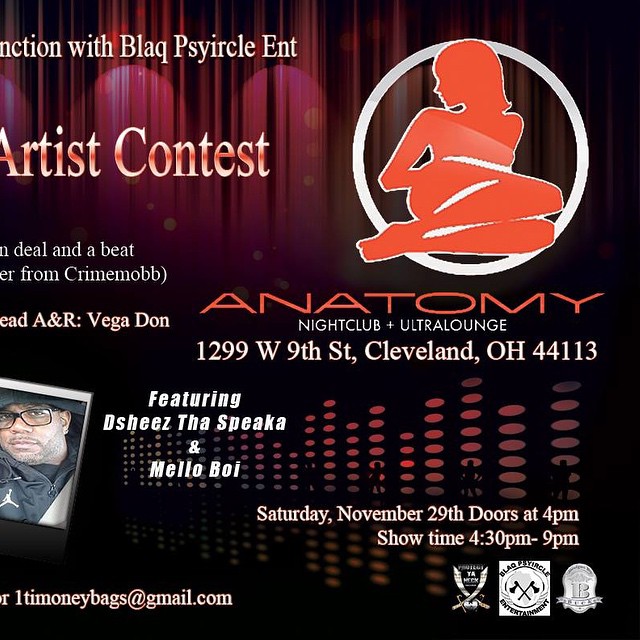This square promotional flyer advertises a music event at Anatomy Nightclub and Ultra Lounge, located at 1299 West 9th Street, Cleveland, OH 44113. The background features a blend of black and dark red, with a digital image of a stage curtain that fades from purple to red towards the right. In the upper right corner, there's a red drawing of a woman lounging and looking over her shoulder, encircled in white. The partially cut-off text in the upper left corner appears to say "junction with Blaq Circle Ent Artist Contest." Below this, in a mix of reddish pink and black text, it mentions "Deal and Beat from Crime Mob" and "A&R Vega Dawn." 
Below the woman's image, "Anatomy" is written in orange, followed by "Nightclub plus Ultra Lounge" in white. The left side features a photo of the event host, a man with glasses and a hat, and below his image is an email address for more information. To the right of his photo, it lists featured artists "D She's, Spica, and Mellow Boy," followed by red dots. In the bottom right corner, white text indicates the event date and time: "Saturday, November 29th, doors at 4, showtime 4:30 to 9." At the very bottom, three logos complete the detailed, vivid flyer.